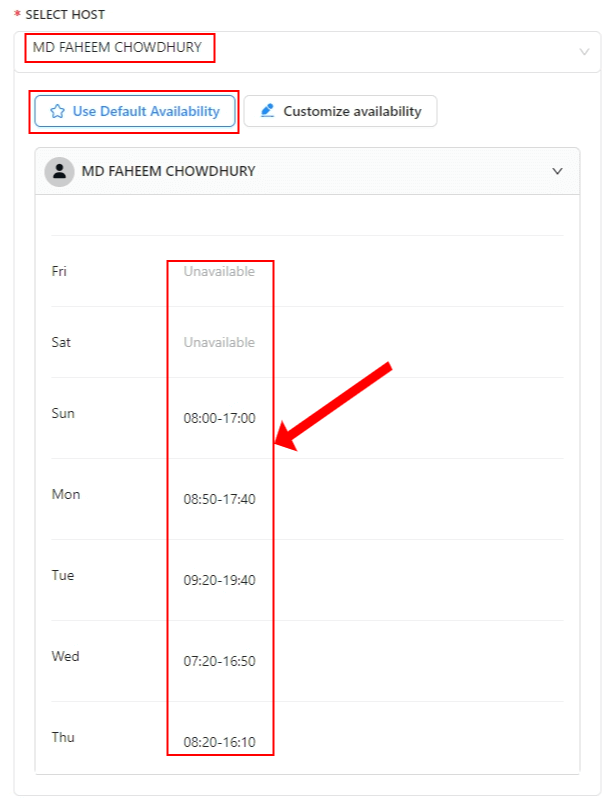The image predominantly features a white background. At the top, there is a small red star followed by the text "SELECT HOST" written in bold, gray capital letters. Below this heading is a white bar containing the name "MDE FAHEEM CHOWDHURY" also in capital letters and gray font, enclosed within a red rectangular outline.

Underneath, there are two outlined sections: the first is a faint red rectangular box containing an inner blue rectangle with a star outline and the text "USE DEFAULT AVAILABILITY" in blue font. Adjacent to this section is an icon of a pencil followed by the text "CUSTOMIZE AVAILABILITY" in a darker font.

Further down, there is a black circular icon depicting a head and shoulders. Next to this icon, the name "MDE FAHEEM CHOWDHURY" is repeated with a small downward-facing arrow on the right side. To the left, a series of abbreviated weekday names are listed in a column: FRI, SAT, SUN, MON, TUE, WED, THU. Each corresponding row indicates availability:
- FRIDAY: UNAVAILABLE
- SATURDAY: UNAVAILABLE
- SUNDAY: 0800-1700
- MONDAY: 0850-1740
- TUESDAY: 0920-1940
- WEDNESDAY: 0720-1650
- THURSDAY: 0820-1610

A red line outlines the "UNAVAILABLE" entries and the schedule for the rest of the week. On the right side, there is a thick red arrow pointing specifically to the Sunday row, aligned down the right side of the schedule, ending just below the "1700" time mark. This arrow highlights an area that seems unusual in its placement.